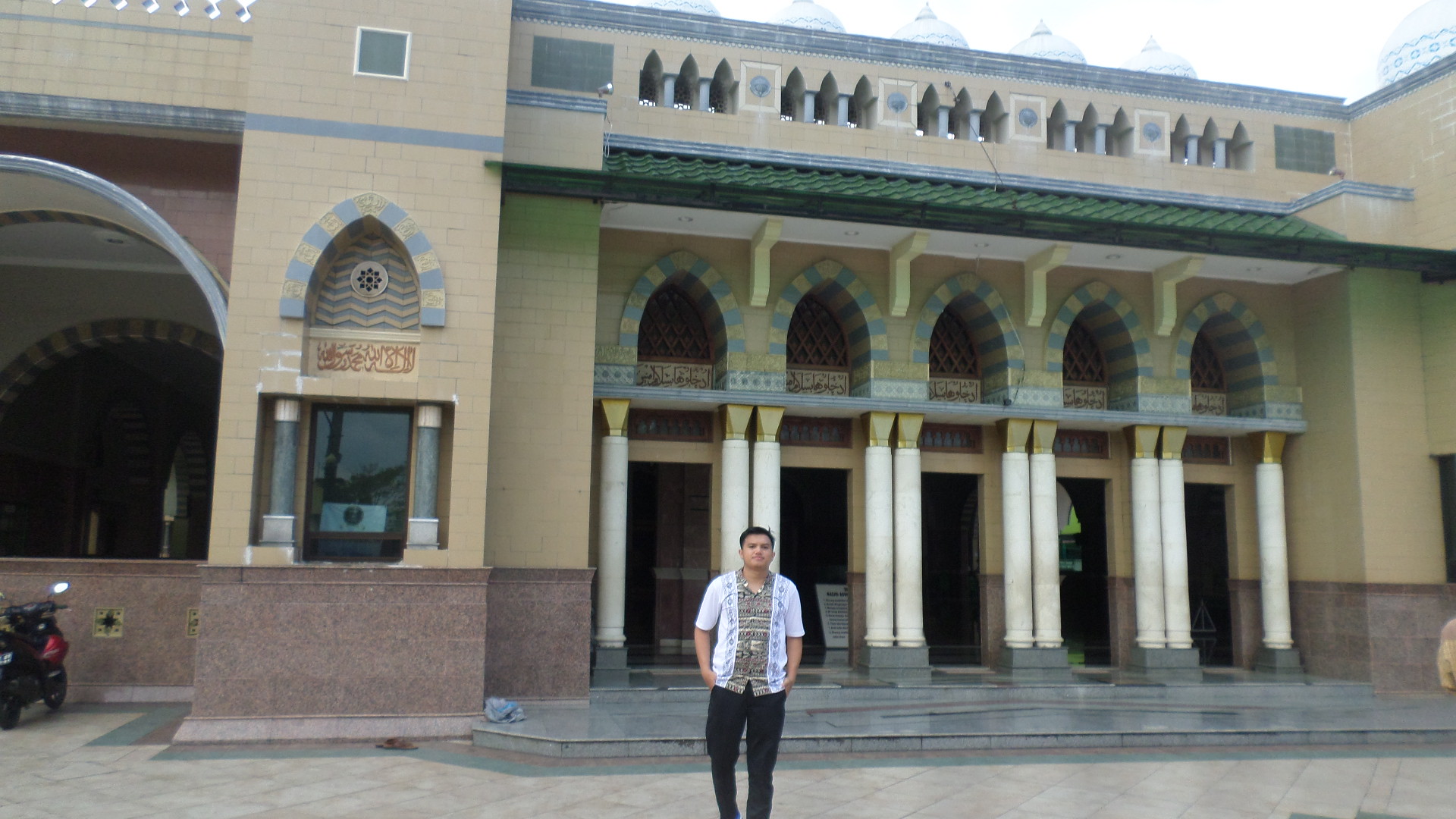The photograph captures a Muslim building bathed in bright daylight, set against a white sky. The structure, which spans the entire width of the image, is characterized by its distinct architectural features. Dominating the center are five archways, each supported by columns and adorned with alternating blue and light green tiles. Above the arches, small openings punctuate the upper section of the beige facade, which is trimmed in blue. To the left of the arches is a large, almost delivery-type entrance, with a niche or window framed by two poles capped in white and resting on square bases. The lower portion of the building is constructed from brown cinder blocks, while the upper area above the arches is painted yellow.

Standing center-bottom in front of the building is a solitary man wearing a white, short-sleeved, open jacket over a colorful, possibly traditional Muslim shirt that reaches his waist. He is dressed in dark pants and has his hands in his pockets, facing the viewer. On the far left, a motorcycle is parked, its right mirror catching the sunlight. This detailed scene, with its vibrant colors and architectural intricacies, provides a rich visual narrative of the setting and the individual within it.